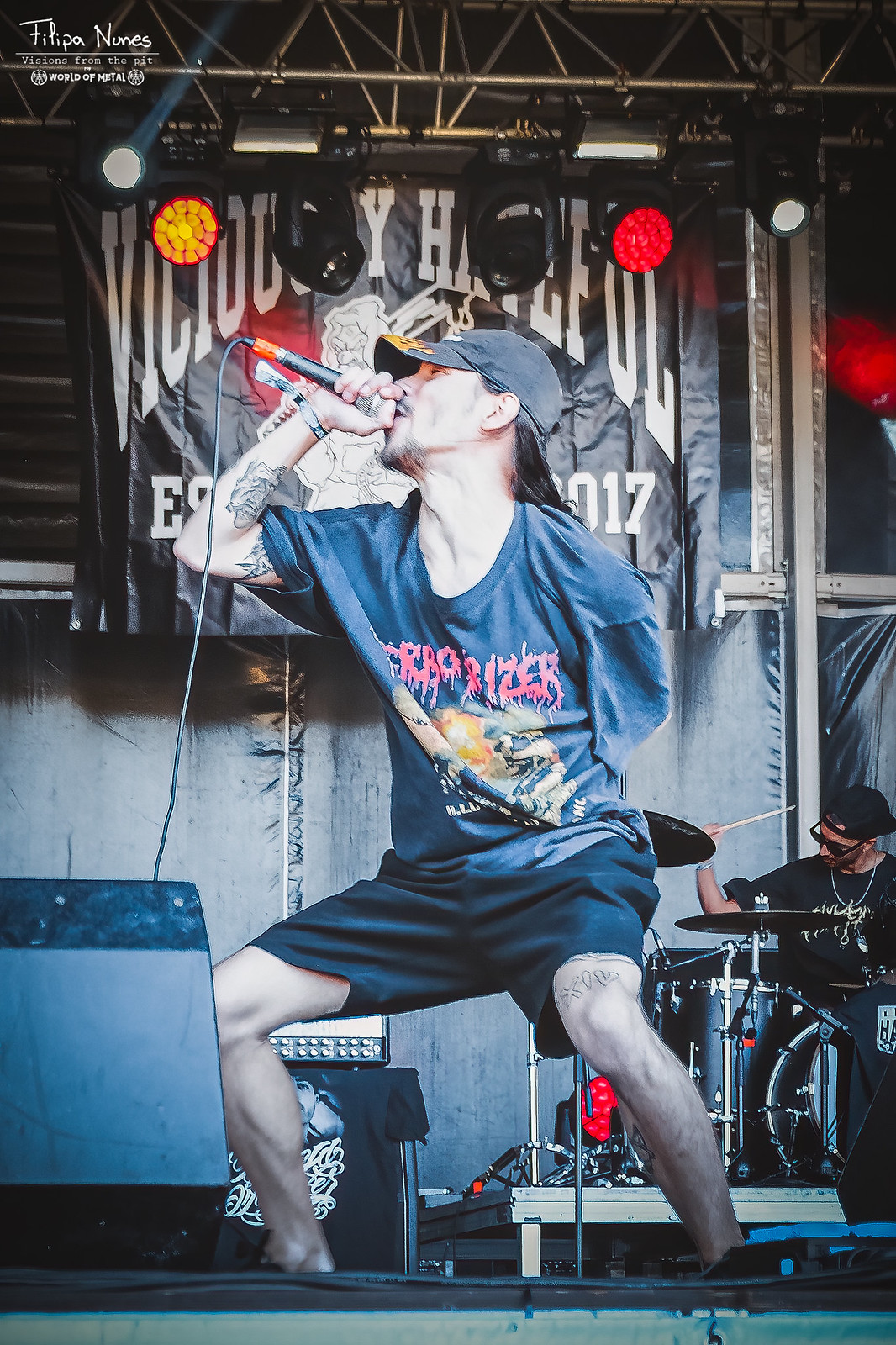In this dynamic photograph, a man passionately sings on stage, fully immersed in his performance. With his knees bent and his head tilted upward, he leans into the microphone that he holds up to his lips. He is dressed in a blue t-shirt adorned with an emblem and unreadable writing, blue shorts, and a gray ball cap with an orange bill. The singer is an amputee, missing his left arm, but this does not diminish his commanding presence. Behind him, bright red and yellow stage lights illuminate a black sign with white lettering that is partially obscured, hinting at the words "viciously hateful" and the year “2017.” In the background to the right, a drummer in a black t-shirt and orange-tinted glasses plays at a full drum set, positioned on a slightly elevated surface separate from the main stage. An amplifier and other stage equipment, including a blue speaker with a dark blue top, are visible in front of the singer, adding depth to the scene. A divider also segments the back of the stage, contributing to the layered and vibrant setting of this captivating performance.